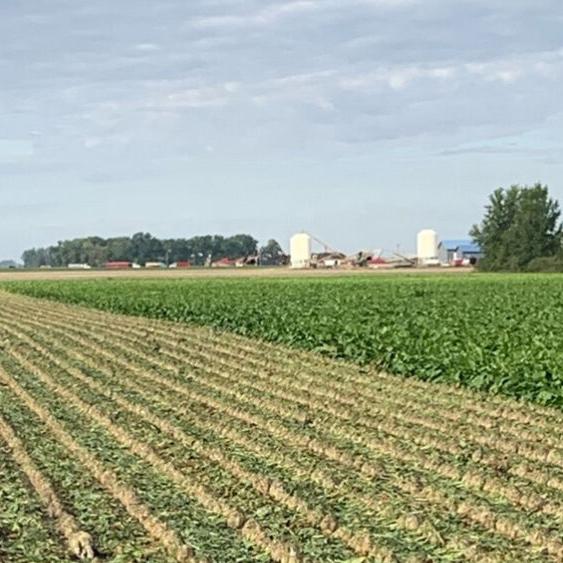This photograph captures a vast expanse of farmland, distinctly divided into sections of harvested and unharvested crops. On the left side, rows upon rows of crops have been meticulously harvested, their remains neatly aligned. In contrast, the right side features lush green plants still standing tall, clearly untouched by the harvester. The field stretches into the distance where a line of vibrant green trees forms a natural boundary. Beyond these trees, two large white cylindrical structures, likely silos or grain bins equipped with augers, stand prominently. Also on the right side are several buildings, including barns with blue roofs, and a prominent large tree adds to the rural aesthetic. In the far background, faintly visible near another stand of trees, are a few trucks, indicating ongoing agricultural activity. The sky overhead is painted with a mix of blue and patches of white clouds, suggesting an overcast yet brightly lit day. The overall scene is tranquil and devoid of any human or vehicular presence, offering a pure and untainted view of the farmland.